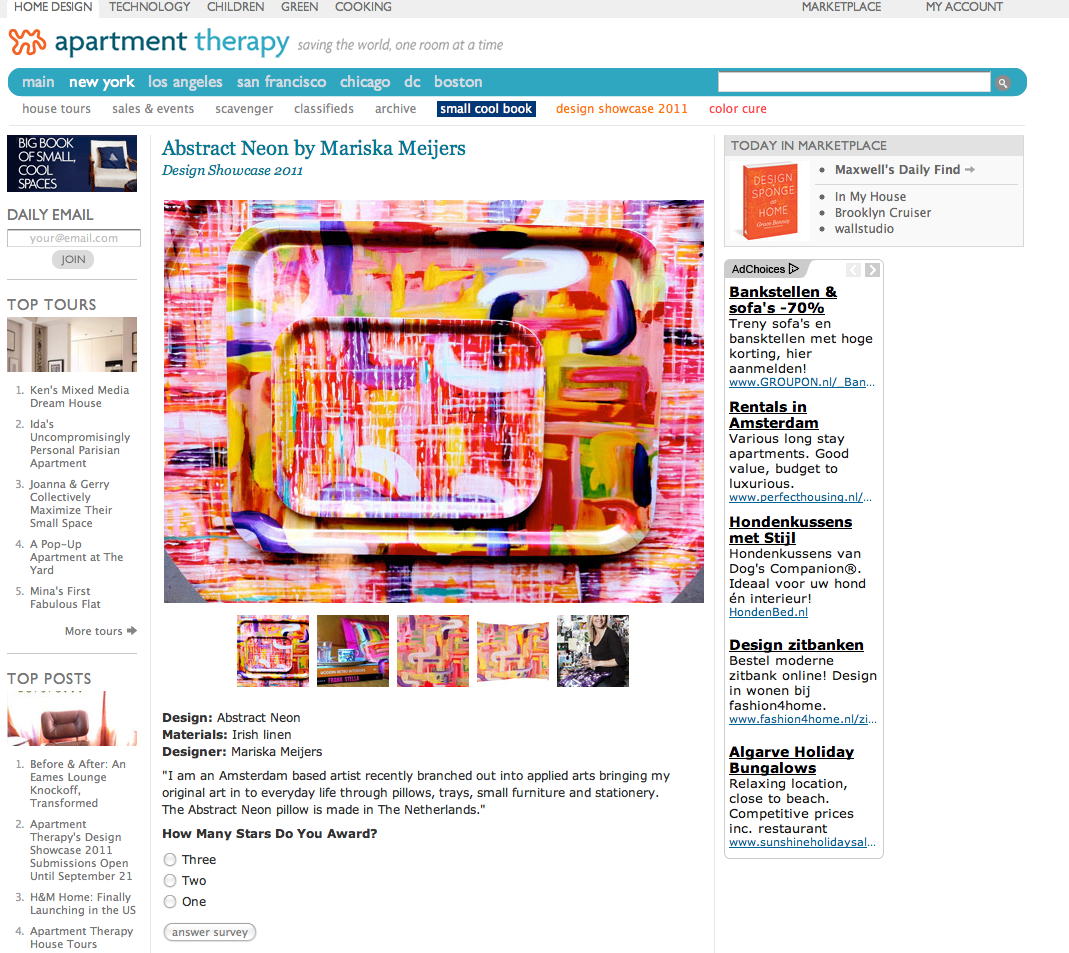Here is a detailed and cleaned-up caption for the image described:

---

An Apartment Therapy webpage showcases an article titled "Abstract Neon by Mariska Meyers, Design Showcase 2011." The centerpiece of the article features a striking photograph of three large trays adorned with vibrant abstract designs. Below this main image, a selection of five smaller pictures is displayed: four capturing similar abstract artworks and the fifth depicting a smiling woman—presumably Mariska Meyers—proudly holding up one of her creations. The accompanying text introduces the "Abstract Neon" series, detailing that the pieces are crafted from Irish linen by Mariska Meyers, an Amsterdam-based artist. It highlights her recent foray into applied arts, where she brings her unique abstract designs into everyday items such as pillows, trays, small furniture, and stationery. Notably, the abstract neon pillow is made in the Netherlands. The webpage is bordered by a green bar at the top, featuring a menu and a search bar, with columns of additional menu items on either side of the article. The right column also contains several advertisements.